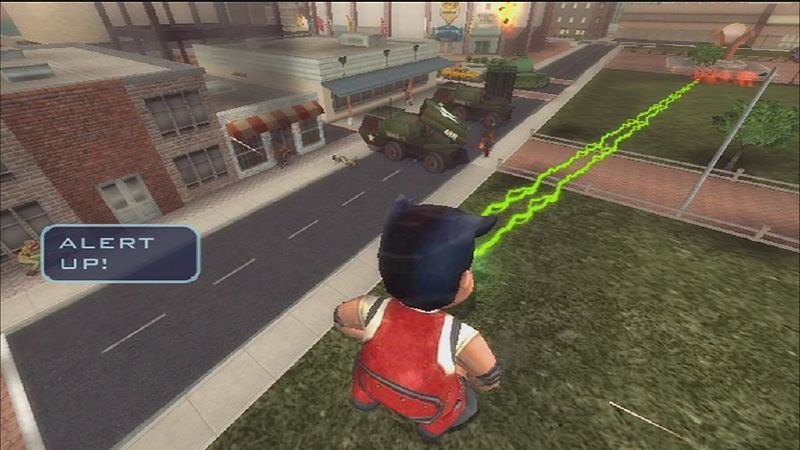Screenshot from a video game depicting a bustling urban environment: On the left side of the image, several buildings resembling shops are lined up with awnings over their entrances, suggesting a marketplace or commercial district. In the background, additional buildings can be seen, adding depth to the scene. The right side features a road flanked by a grassy area with trees and a walkway, providing a touch of nature amidst the urban setting. Centered on the road are military vehicles, including missile launchers and a tank, indicating a possible confrontation or defensive scenario. In the lower right corner, a character with black hair is visible from behind. He is outfitted in a white shirt paired with red overalls and is dramatically shooting green plasma rays from his eyes, adding an element of sci-fi or fantasy to the scene.